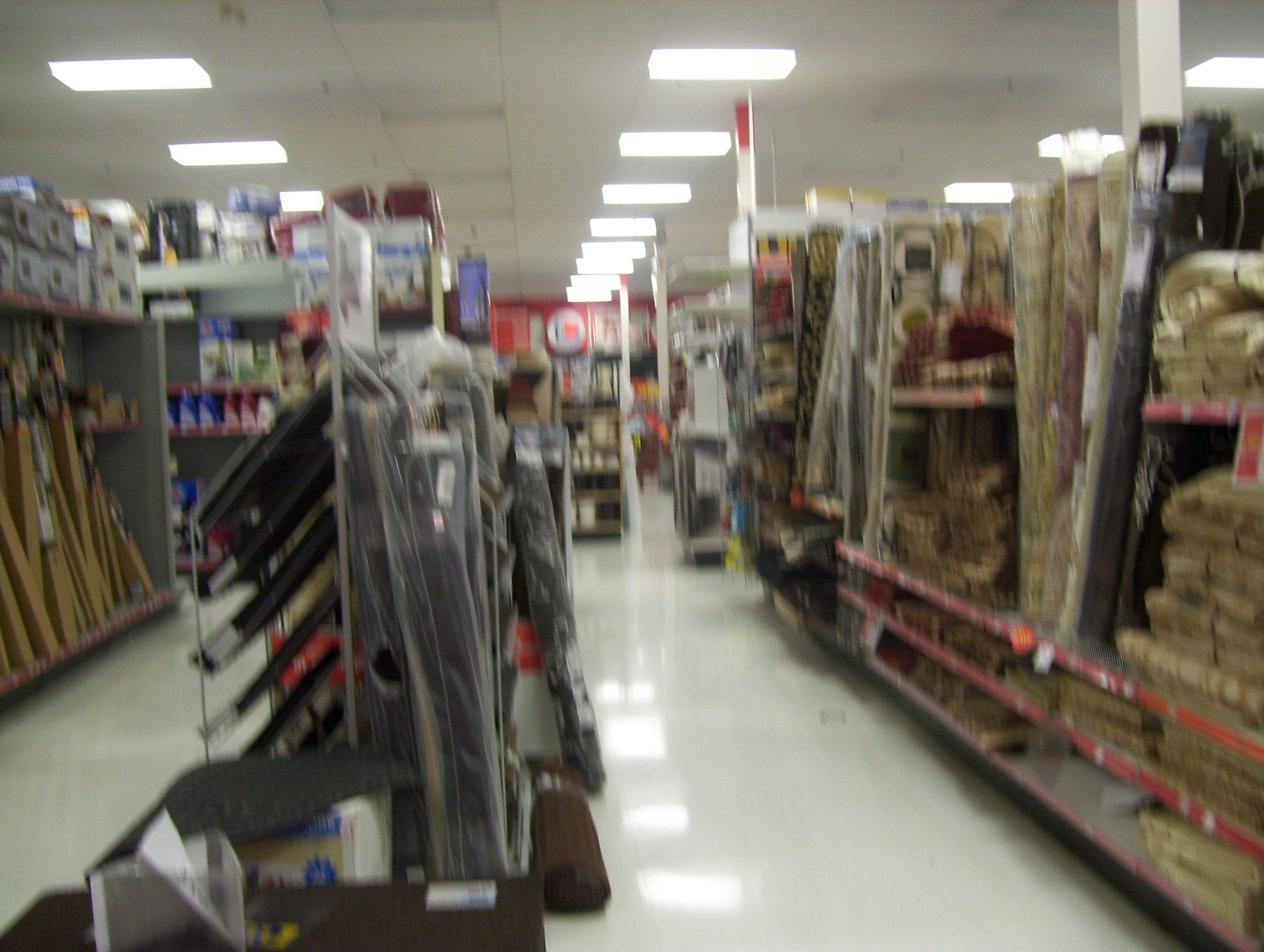The image depicts the inside of a home improvement store. The scene is blurred but provides a clear view of two central aisles. On the right, there is a collection of large, rolled-up rugs secured by two red bars on a shelf, preventing them from toppling over. Smaller folded rugs, shaped into squares, are also visible next to the rolled ones. The left side of the main aisle features various home goods, including items that are difficult to identify due to the blurriness, but wooden planks are distinctly visible. Further down the main aisle, vases and pots can be seen, indicating an extensive selection of home decor and improvement items. 

The store's design includes white, warehouse-style ceiling tiles with integrated artificial lighting that reflects off the white concrete floor. Although the store's dominant color appears to be red, giving it a distinctive theme, it does not distinctly resemble any particular well-known retail chain. The overall ambiance suggests a spacious, well-lit, and organized environment tailored for a variety of home improvement needs.